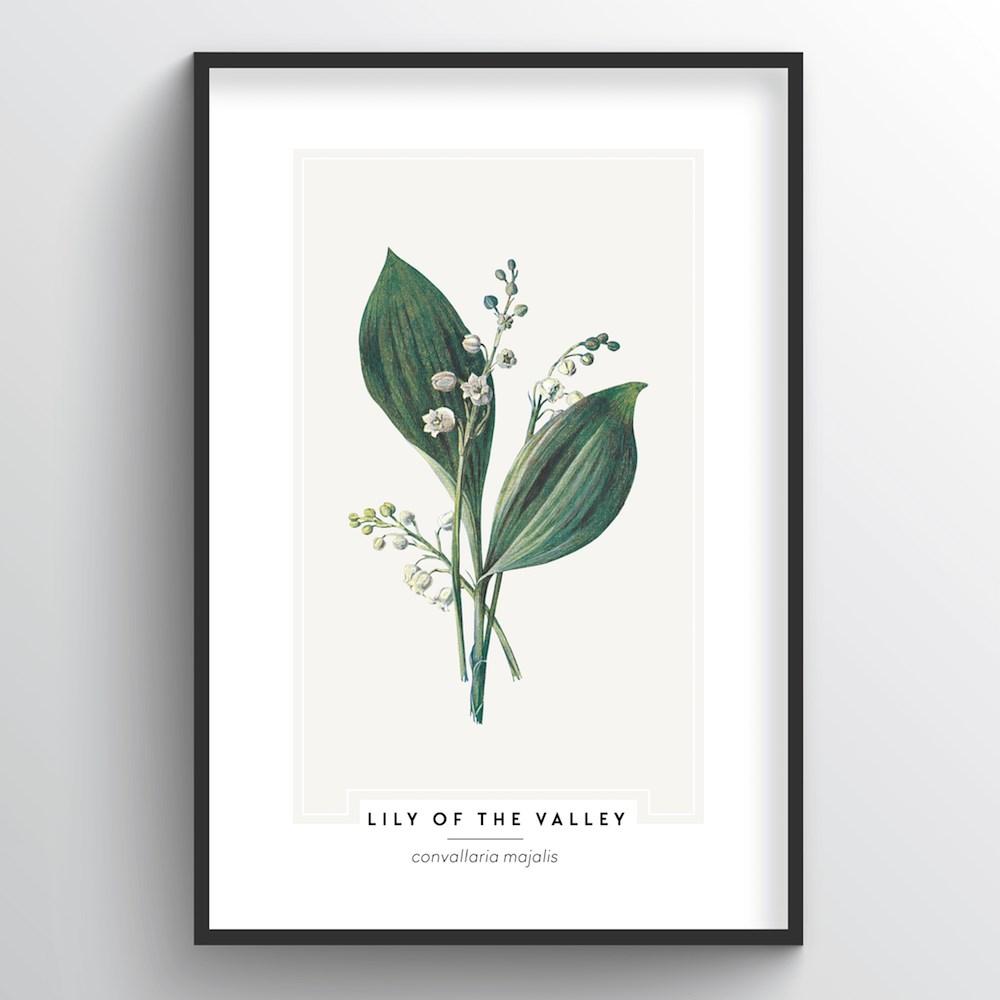The image depicts a framed black and white print of a Lily of the Valley against a white wall. The frame is thin and black, with a white mat surrounding the artwork. The print features an elegant and simple botanical illustration of two large green leaves and three stems of white bell-shaped flowers, identified as Lily of the Valley. Beneath the image, the common name "Lily of the Valley" is accompanied by its Latin name, "Convallaria majalis," providing both aesthetic appeal and educational value. The lighting in the room creates a gradient shadow on the wall, adding depth and highlighting the peaceful simplicity of the piece.